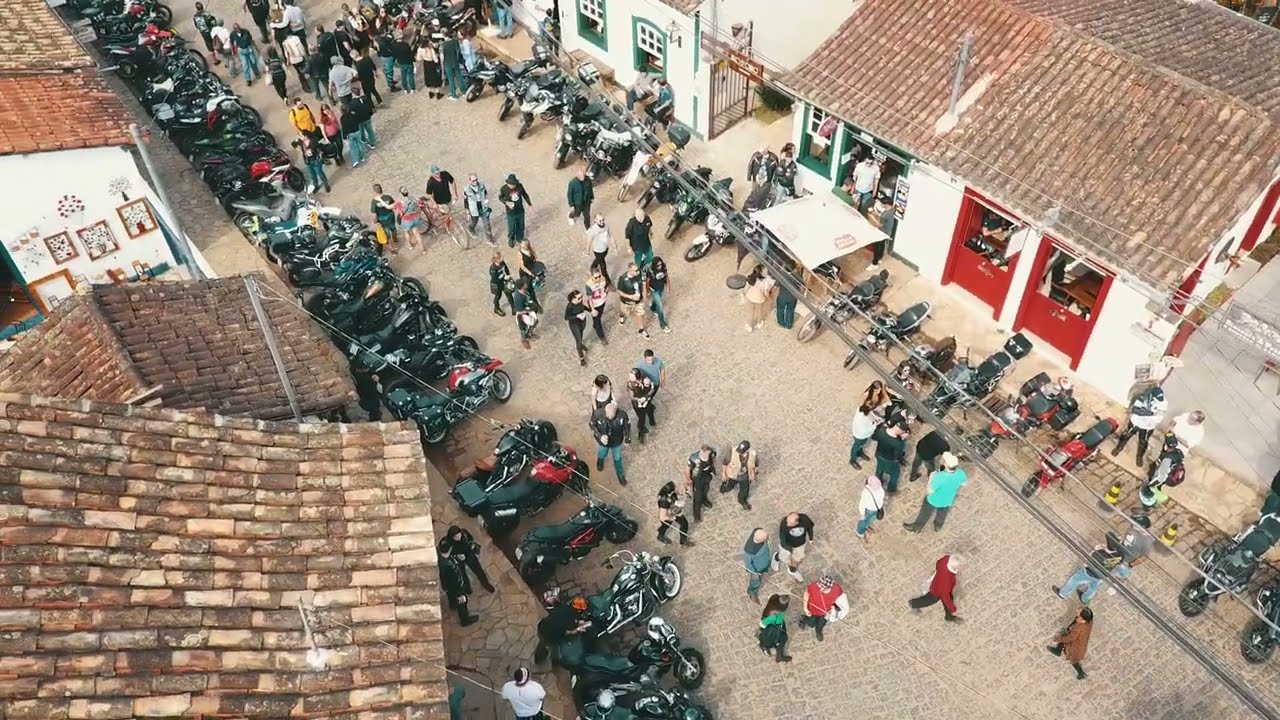This detailed aerial photograph, taken during the daytime, offers an expansive view of a street made of light brown cobblestones. The street spans diagonally from the bottom right to the upper left of the image. On both sides of the street, motorcycles are neatly lined up, creating a striking visual that suggests a significant gathering of enthusiasts, possibly at an event like the Sturgis Motorcycle Rally in Montana. The rows of parked motorbikes extend the full length of the street, bordered by buildings with mottled brown clay stone roofs. On the right, buildings feature open window counters, hinting at shops with people engaging through the windows. The left side showcases similar buildings, with indistinct frontages due to the aerial perspective. Pedestrians fill the center of the street, freely walking and mingling among the bikes, reinforcing that the area is closed to traffic. Additionally, power lines run down the center of the street, paralleling the pedestrian pathway, further emphasizing the organized chaos of this bustling street scene.